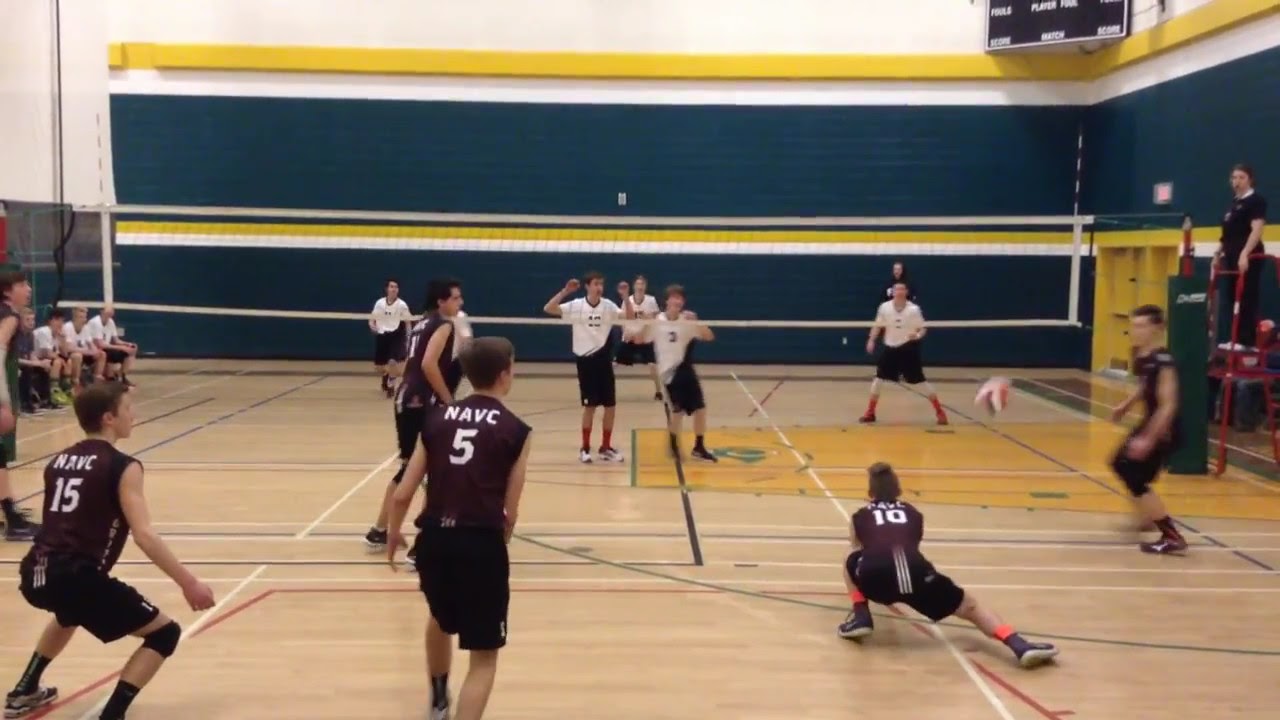The image captures an intense indoor volleyball game, likely at a school gymnasium. Two teams are mid-play, divided by a central net. The team on the left side of the net is dressed in white t-shirts and black shorts, with most players wearing a mix of black or red socks. The opposing team on the right wears burgundy t-shirts with black shorts, and their jerseys are emblazoned with numbers such as 5, 10, and 15. One notable player from the burgundy team is crouched down, poised to receive the ball, as everyone's attention is focused on him. The gym features dark blue walls adorned with yellow stripes, adding a vivid backdrop to the scene. There is a referee visible on the right side of the image, while some substitute players from the white-shirt team are seated on the bench to the left. The letters "NAVC" can be seen printed on the back of the players’ jerseys, indicating likely team initials or a school abbreviation. The overall atmosphere reflects the competitive spirit of a school sports event, with both teams striving to gain the upper hand.